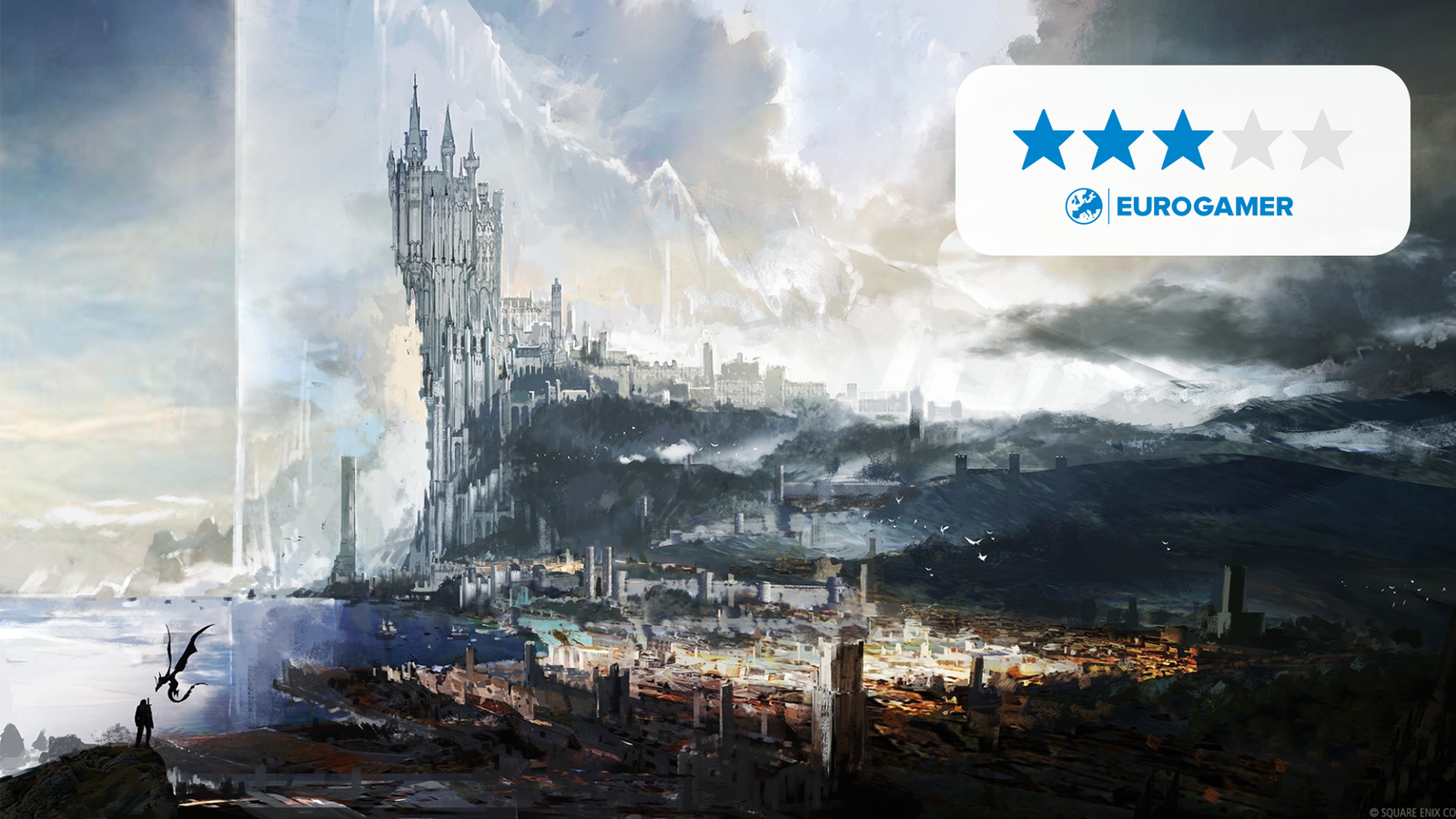This image, likely a screen capture from a video game reviewed by Eurogamer (rated 3 out of 5 stars), depicts an intricate artwork of a fantasy city set in a valley under a cloudy sky. In the background, a majestic, silver-turreted castle rises along a mountainous ridge to the left. Below, the city shimmers with contrasting dark and bright elements, highlighted by scattered golden hues. In the lower-left corner, a lone figure stands on a rocky outcropping, observing the scene. Near this person, a small, thin-bodied dragon with long wings is in flight, adding to the mythical ambiance. The city's bright central lights contrast with the predominantly darker tones of black, gray, and light blue sky, completing this vivid, surreal illustration.